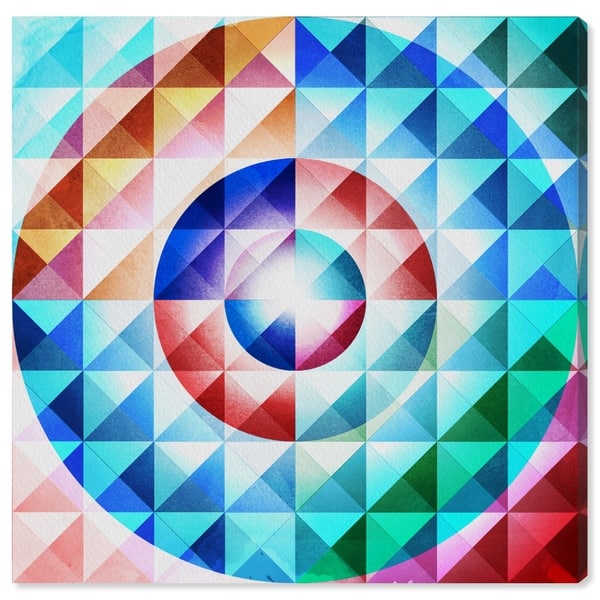This image is of a vibrant geometric artwork, presumably a painting on a 3D canvas. It primarily consists of numerous small squares, each divided into four triangles, creating a diverse collage of colors. These triangles vary in hues, ranging from reds and yellows to blues, pinks, teals, oranges, and greens. The arrangement of the colored triangles gives the illusion of a series of concentric circles. A large circle spans edge to edge of the painting, within which smaller circles nestle, culminating in a bright, almost blinding white center, reminiscent of an eye or a radiant light source. The visual complexity, with overlapping shapes and the interplay of colors, evokes a kaleidoscopic effect, offering a mesmerizing and somewhat perplexing experience. The entire piece presents a blend of geometric precision and vibrant chaos, set against a plain white background, drawing the viewer's eye towards the luminous core of the composition.